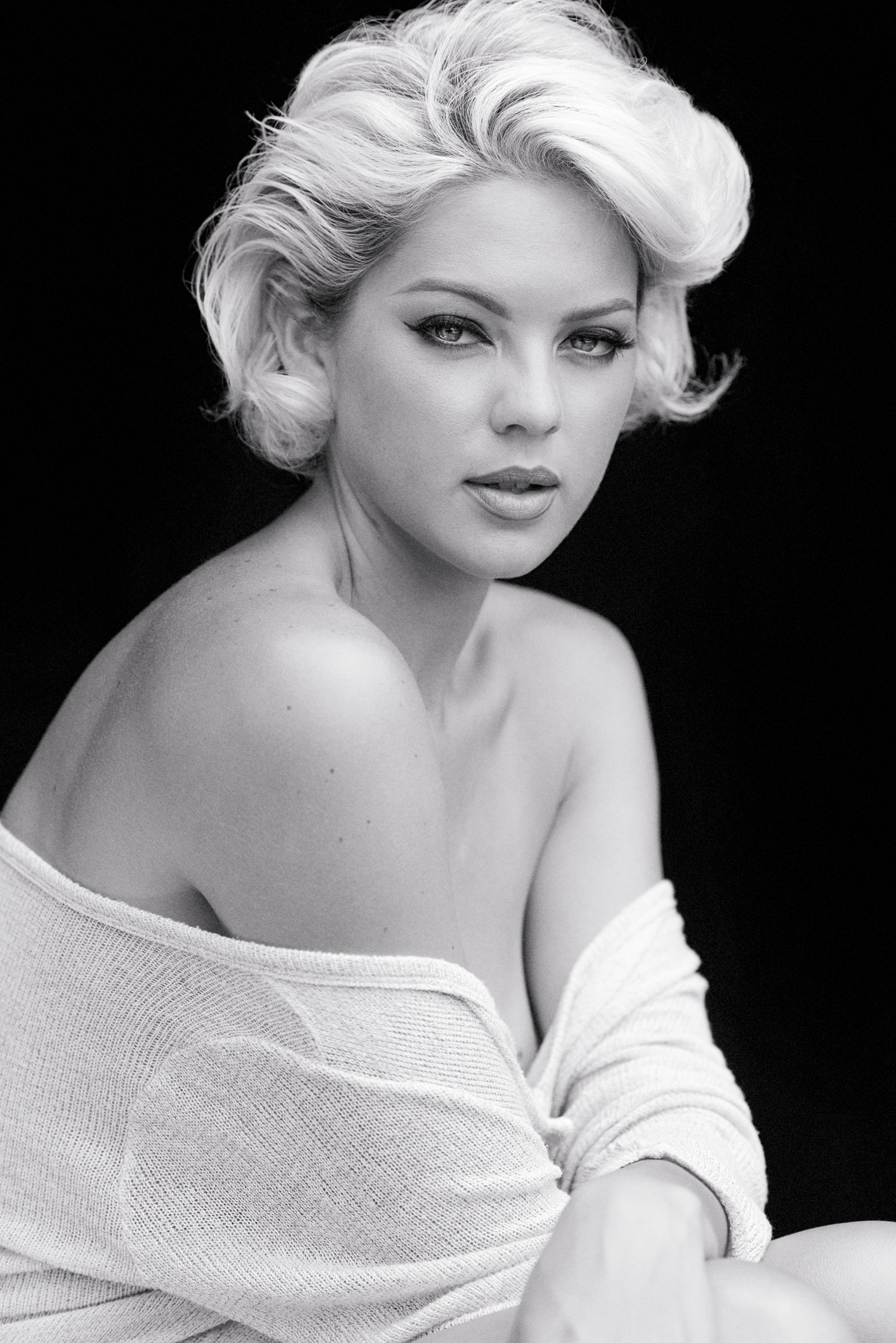This striking black and white photograph depicts a captivating woman with short, platinum blonde hair styled stylishly back, parted slightly to the side, and slicked behind her ear. Her hair reaches the beginning of her jaw and has a smooth, voluminous texture. Her makeup accentuates her features, with lined lips, winged black eyeliner, and mascara highlighting her expressive eyes. She gazes directly into the camera, creating an intense, intimate connection with the viewer.

The woman, who appears to be Caucasian, is seated with her arms crossed over her knees. She is draped in a sheer, meshy top that wraps around her upper arms, shoulders, and triceps, leaving her upper back and shoulders bare. The top modestly covers her chest as it cascades stylishly to her elbows and is tucked into her lap. Her relaxed pose and the placement of her arms suggest a sense of poise and grace.

The composition features a pure black backdrop, which contrasts sharply with her light-colored hair and fair complexion, drawing the viewer's attention entirely to her. The subtle details and textures in the image, from the delicate fabric of her top to the contours of her hair and makeup, together create an evocative, timeless portrait.